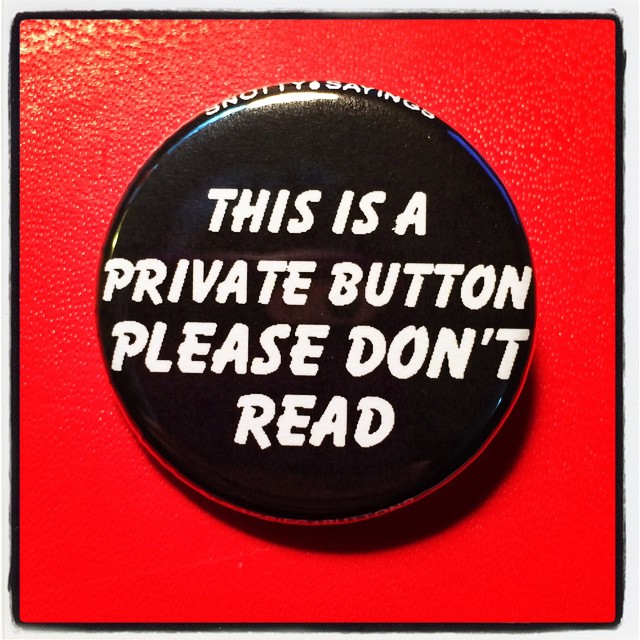The image depicts a textured red square with a slightly uneven paint application, suggesting it may be painted on a concrete wall or a similar rough surface. The red square is bordered by a black edge. At the center of the red square, there is a prominent black circular button featuring large, white, all-capitalized text that reads, "THIS IS A PRIVATE BUTTON. PLEASE DON'T READ." The text adds a humorous touch, implying an ironic invitation to read despite its warning. Above the button, a smaller inscription in white reads "SNOTTY SAYINGS." The black button casts a noticeable shadow on the red background, creating a crescent moon shape on the lower right side. The background hints at additional colors and textures, with some blue tones appearing towards the top and red tinges at the bottom. There's also a mention of gold flecks or dots near the upper left-hand corner, adding further detail to the red square's appearance.